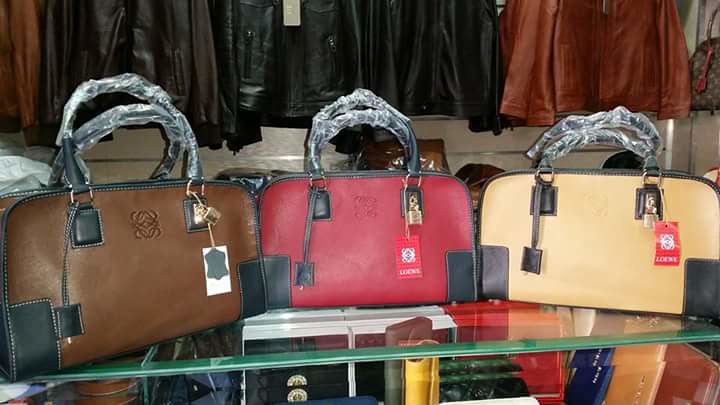This photograph captures a vibrant display of designer handbags and colorful wallets in what appears to be a high-end leather store, evoking a sensory impression of rich leather aroma and soft textures. Positioned atop a sleek glass display cabinet are three meticulously crafted leather bags with slightly rectangular shapes and black handles wrapped in protective plastic. Each handbag features distinctive black trim and a hang tag advertising the manufacturer. From left to right, the bags are: a dark brown bag with a black border, a deep red bag with black trim, and a pale yellow bag also adorned with black detailing. Beneath these handbags, the cabinet houses a delightful assortment of colorful leather wallets in shades of red, blue, brown, beige, green, and yellow. Behind the display, an array of leather jackets in black, brown, tan, and reddish-brown hangs, adding to the luxurious and sophisticated ambiance of the store.